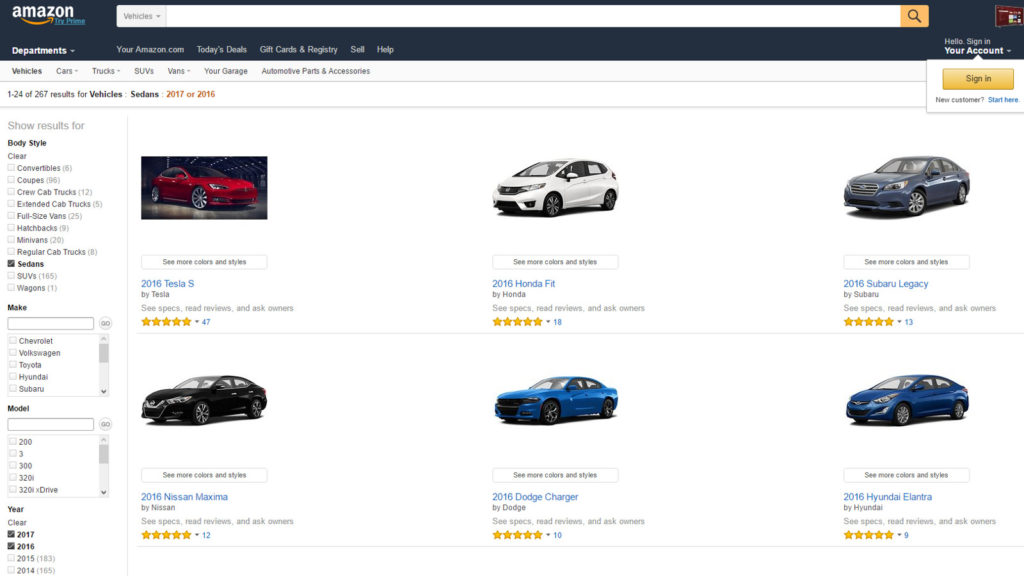This detailed caption reads:

"A highly detailed photographic image showcases an Amazon web page prominently featuring the Amazon logo on the top left corner, encompassing the white Amazon text, the signature yellow arrow, and 'Prime' indicated in blue. At the top of the page is a web bar with a search engine, including a magnifying glass icon and a yellow 'Sign in to your account' button. The web page displays search results for vehicles, highlighting various models from the year 2016. Visible on the screen are a red Tesla Model S with a five-star rating, a white Honda Fit with a five-star rating, a blue Subaru Legacy with a five-star rating, a Nissan Maxima with a five-star rating, an electric blue Dodge Challenger with a five-star rating, and a blue Hyundai Elantra with a five-star rating."